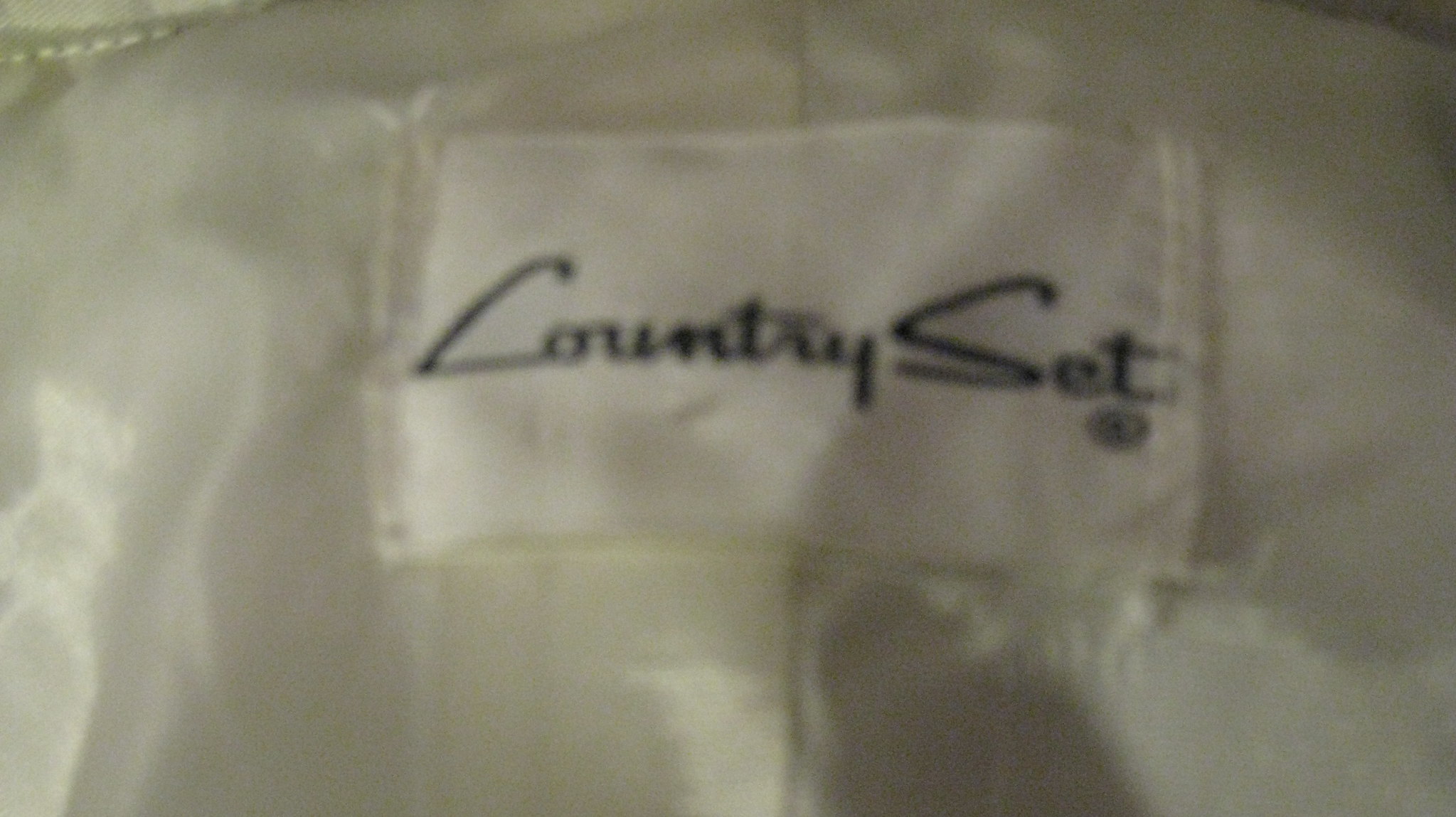This photograph captures a fabric tag meticulously sewn onto a piece of smooth, white satin polyester fabric. The fabric itself glistens with a subtle sheen, suggesting its luxurious texture and quality. Both the tag and the stitching used to affix it blend seamlessly into the fabric, as they are also white. This monochromatic theme creates a uniform, elegant appearance. The tag, crafted from similarly white fabric, features the words "Country Set" elegantly printed in black script, indicating that this piece is part of a set of sheets. The thoughtful craftsmanship and refined details underline the high quality and sophistication of the bedding.